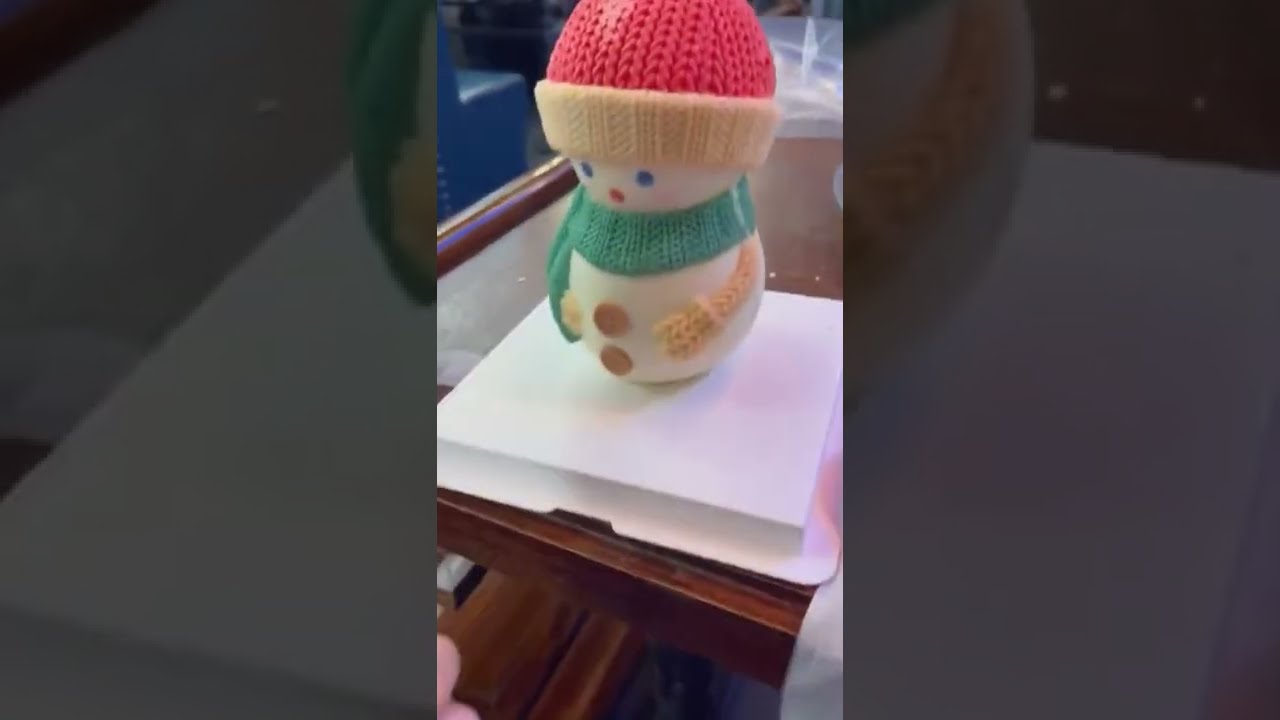The image features a close-up of a small, decorative snowman figurine, reminiscent of Christmas blow mold decorations often displayed on lawns. The snowman is situated on a white, square platform, which rests on what appears to be a brown wooden table with dark brown trim. The table itself might have a glass surface. The snowman is adorned with bright blue eyes, represented by two small blue dots, and has a round red mouth or nose. It wears a charming red knit hat with a cream-colored band and a cozy green scarf draped across its front. The snowman’s arms are beige or tan, ending in cream-colored mittens. Its body showcases two brown buttons on its front. The background is somewhat blurred and includes indistinct items, possibly a blue chair and some sparkly elements in the upper right corner. There’s also a hand or fingertip visible at the bottom left edge of the image. Additionally, the photograph is artistically divided into three sections, with the central part displaying the full snowman figure, flanked by darker, blown-up segments of the figurine and table on the left and right sides.